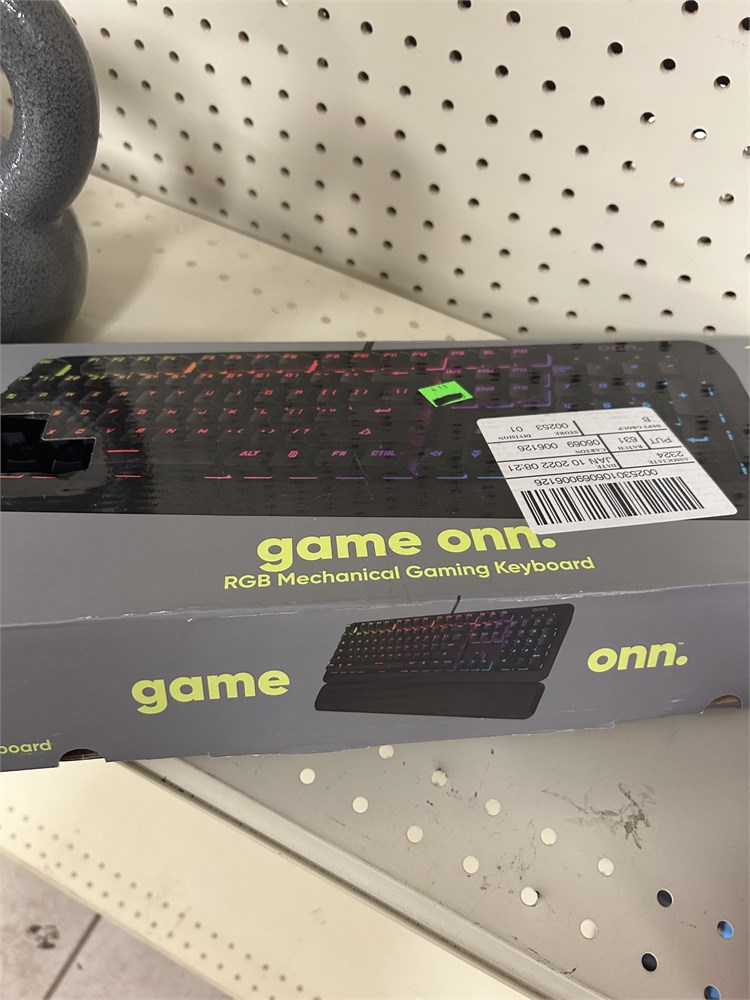In this image, a boxed "Game On RGB Mechanical Keyboard" is prominently displayed on a store shelf, likely at a discount store or thrift shop such as Goodwill. The keyboard is housed in a rectangular, gray box adorned with bold, yellow lettering that reads "Game On RGB Mechanical Keyboard." The box features a vivid illustration of the black keyboard, which is illuminated by colorful RGB LED lights on the keys, emphasizing its gaming-oriented design.

The packaging has two stickers: a small green sticker that seems to indicate the price and a larger white sticker with various numbers and other details, possibly indicating shipping or stock information. The item is positioned on a metal rack characterized by a pattern of multiple small holes, typical of store shelving units.

In the background, to the left of the keyboard box, part of a gray kettlebell is visible, though it is partially cropped out of the frame. The lower left corner of the image reveals a small section of tiled flooring, adding to the context of the store environment. The photograph focuses mainly on the keyboard box, suggesting that it was taken either to highlight the product for potential buyers or to share details of the item with someone else.